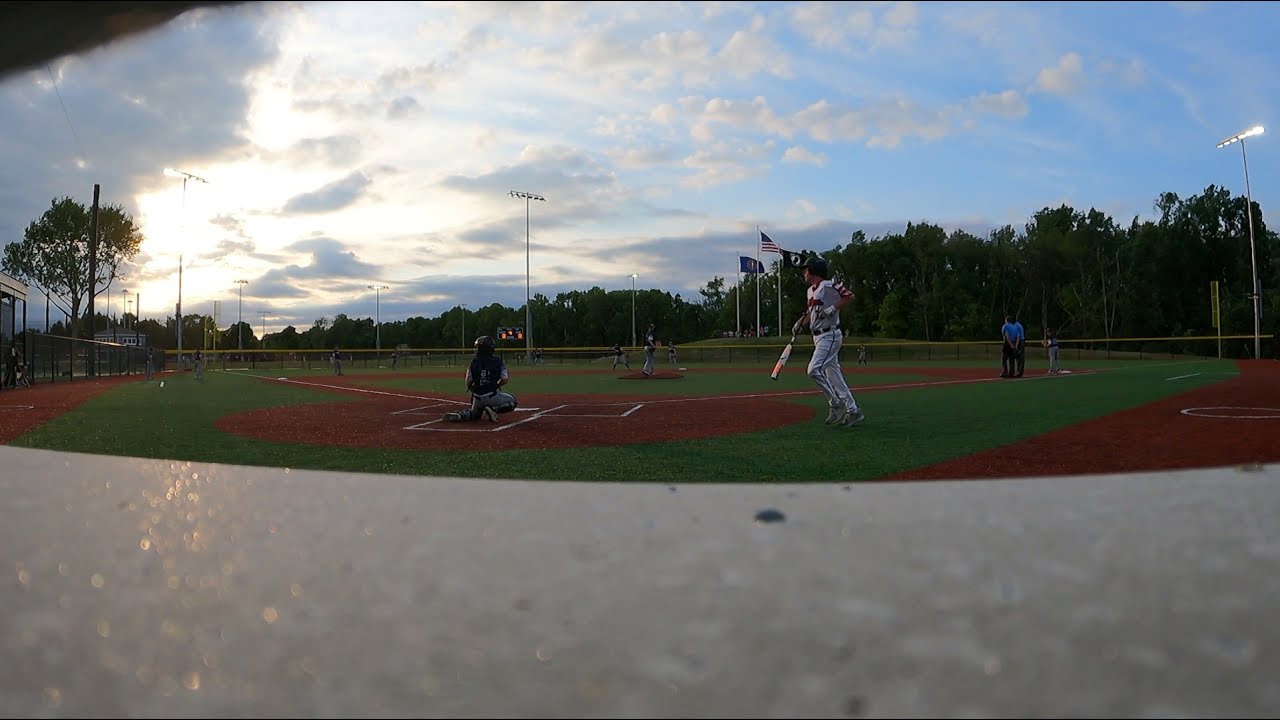In this image, we see a detailed scene of a baseball game unfolding on a field framed by trees under a setting sun, with the sky showing a vivid blue adorned with clouds. Central to the photo is a male player, outfitted in a black helmet, gray shirt, and white pants, walking to the batting area. In his right hand, he clutches a baseball bat with a black handle and an orangey bronze lower half leading to a white upper half. He's approaching the plate, where a catcher, geared in all black protective equipment and helmet, is already in position. On the pitcher’s mound, a player dressed in a black shirt and light gray pants prepares to pitch, looking to the right. Nearby, another player mans first base while two umpires in blue shirts stand close by, with other individuals near second and third base. The photo lacks visible stands or spectators, possibly due to its angle, which suggests it might have been taken through a portion of a fence, evident by some obstructions at the bottom of the image. The sunlight filters through from the center-left, casting a gentle golden hue across the scene, indicating the game is either ongoing or about to start.